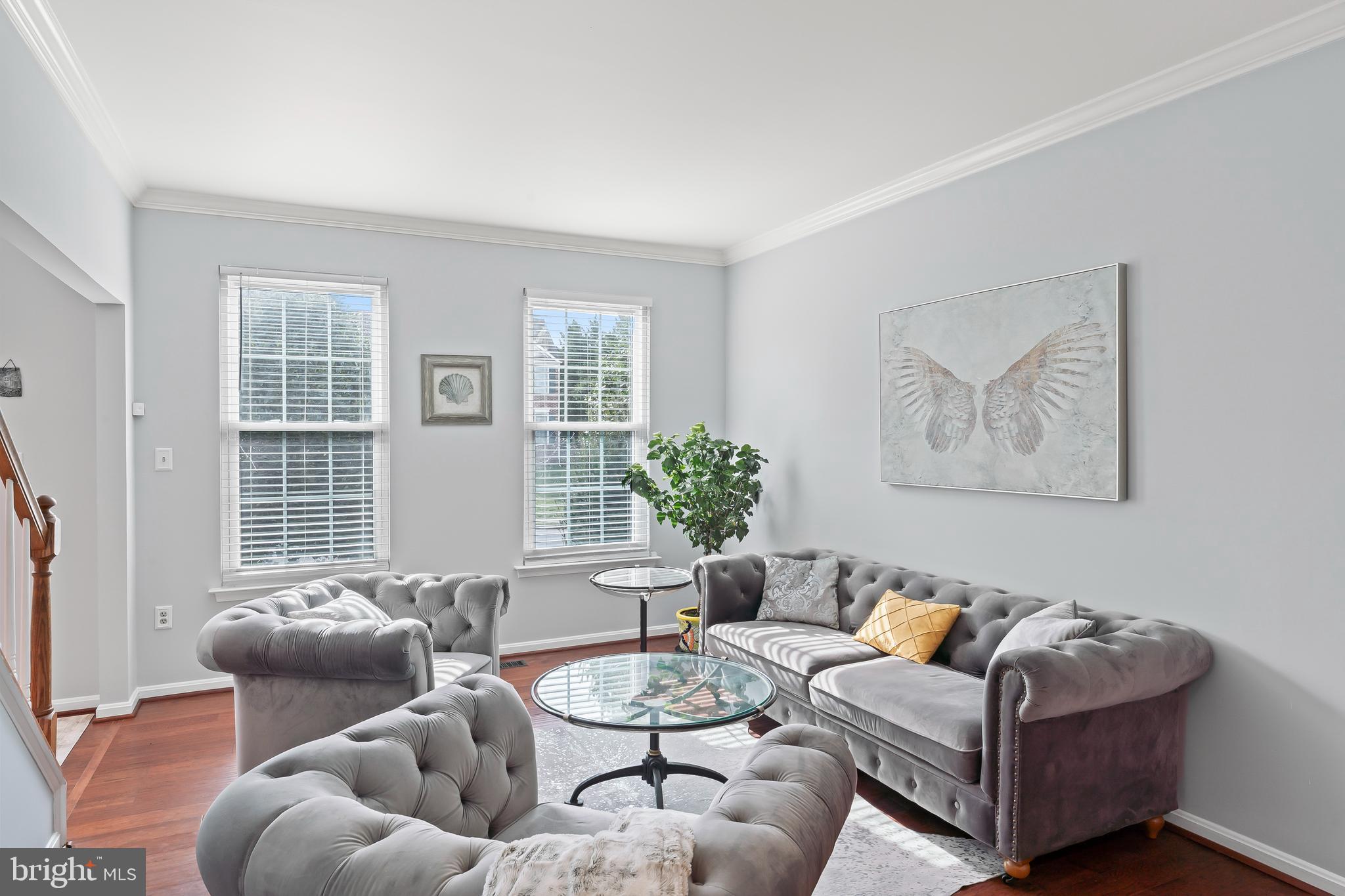This detailed image depicts a sophisticated living room with a predominantly gray color scheme, featuring sleek design elements and stylish furnishings. The room has gray walls with a white ceiling and white border trim. On one side, there are two long rectangular windows with white blinds. Adjacent to the windows, there is a gray-toned painting of a butterfly, complemented by a smaller picture of a gray shell set against a white background.

Central to the room is a seating arrangement consisting of a large gray velvety sofa and two matching tufted chairs, all adorned with various gray pillows and a distinctive orange pillow at the center of the sofa. These pieces are positioned around a circular glass coffee table and a matching glass end table with black stands. 

A plush white carpet with gray accents lies on the polished brown wooden floor, adding to the room’s cozy ambiance. In the corner by the sofa sits a green indoor plant housed in a colorful orange and black flowerpot, providing a touch of natural vibrancy.

Additionally, there is a staircase to the left with white railings and a brown wooden handrail, enhancing the elegance of the setting. Electrical switches and plug areas on the walls are white, maintaining a clean and cohesive look.

The whole scene is completed by the presence of a subtle watermark indicating "bright MLS," suggesting a real estate listing, with white text on a gray background featuring an orange line through the letter 'T'.